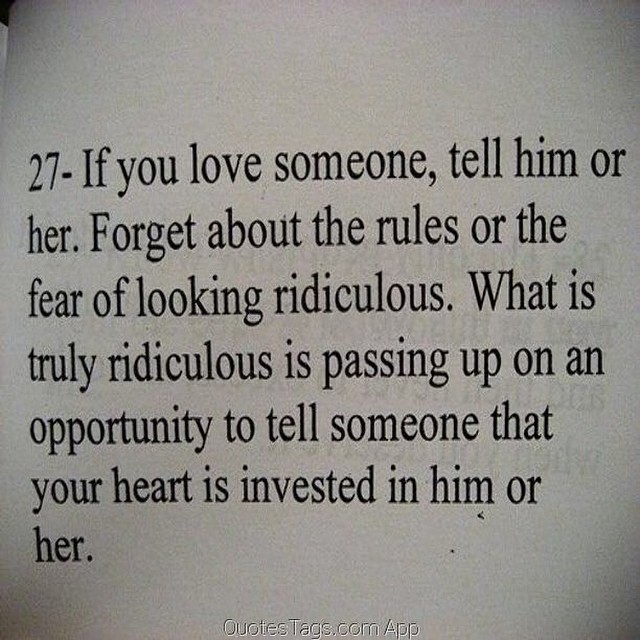The image displays a close-up of a sign or an excerpt from a book with a motivational quote. The background is a grayish-white tint with a darker edge on one side, providing a subtle contrast to the black Arial-style font text. The passage reads: "27. If you love someone, tell him or her. Forget about the rules or the fear of looking ridiculous. What is truly ridiculous is passing up an opportunity to tell someone that your heart is invested in him or her." At the bottom, there is a faint embossed white text, indicating the source as "quotetags.com app". This detailed presentation combines the prominent elements of both descriptions, highlighting the visual and textual components comprehensively.